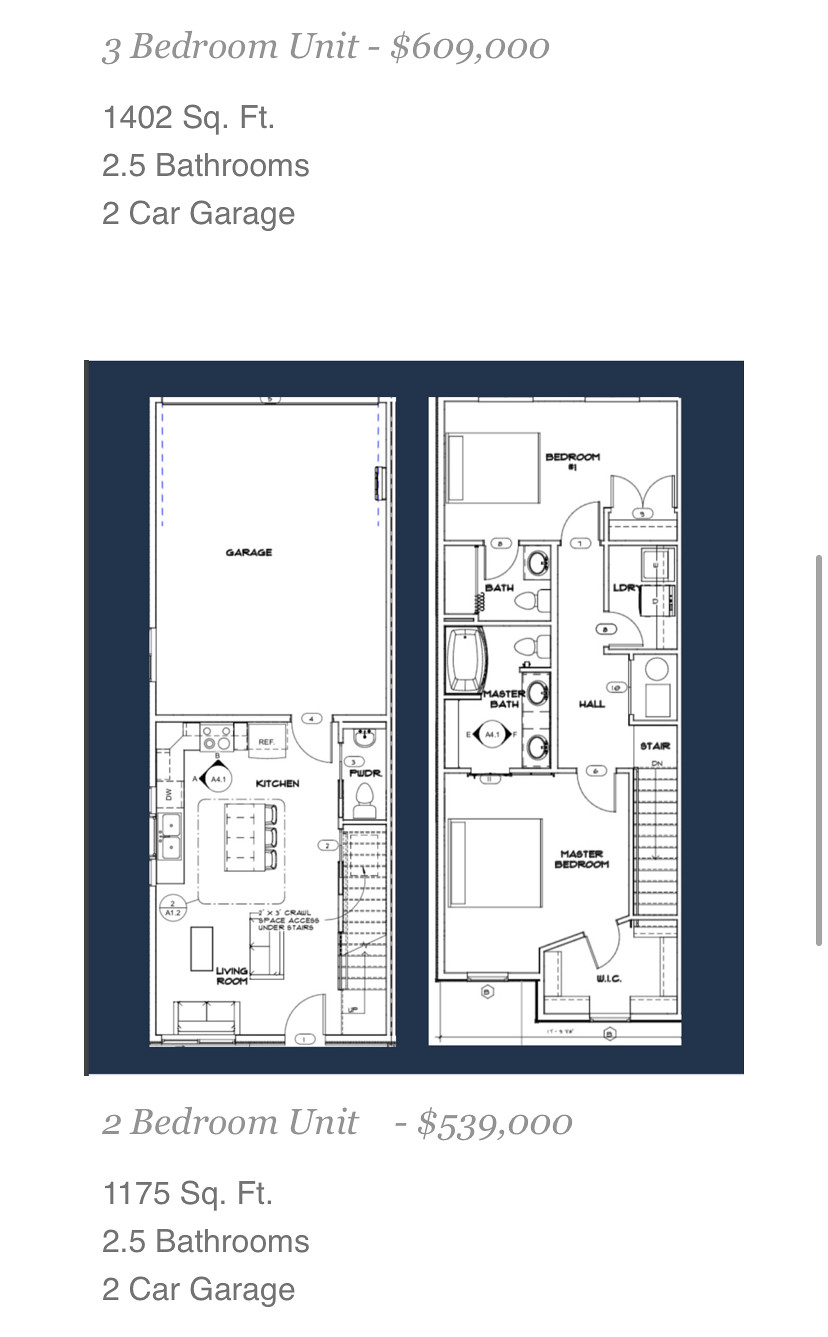This photograph depicts a detailed diagram of an apartment's floor plan. The background of the image is dark, emphasizing the black and white design of the floor plan itself. Text at the top of the photograph initially describes the specifications of a three-bedroom unit, listing a price of $609,000 for 1,402 square feet of space that includes two-and-a-half bathrooms and a two-car garage. Below this text, the diagram appears to pertain more accurately to a two-bedroom unit, as indicated by additional text specifying a price of $539,000 for 1,175 square feet. This unit also features two-and-a-half bathrooms and a two-car garage. The floor plan is detailed and clearly shows a two-story layout, including the placement of the garage.